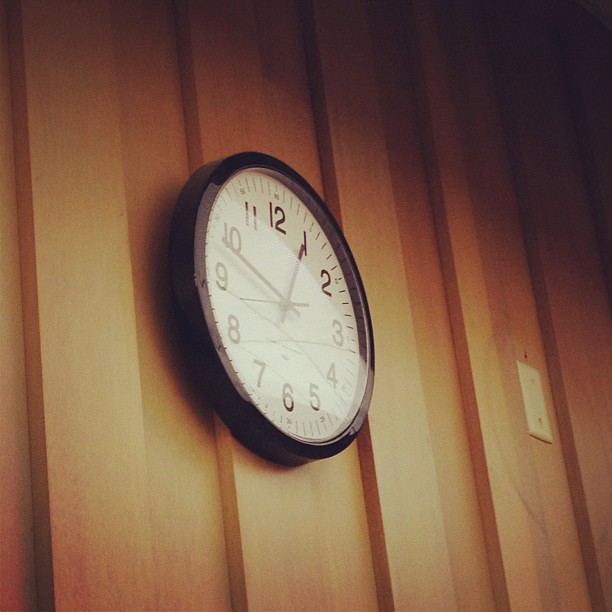The photograph captures a wall-mounted clock within a room with distinctive wooden wall paneling. The wooden wall consists of alternating vertical beams, some protruding and some recessed, giving it a textured appearance in light brown hues. The clock, positioned slightly left of the center, features a plain design typical of office or classroom settings. It has a black, likely plastic casing with a glass cover and a white face adorned with black numbers from 1 to 12. Thin black lines mark the minutes between the numbers. The image is taken from a side view, revealing some context of the room's ambient lighting, which is quite dark, particularly at the top right and bottom left corners, suggesting it might be night. To the far right of the image is a rectangular white plate that appears to be an unusual mount, possibly for future installations, rather than a conventional light switch.